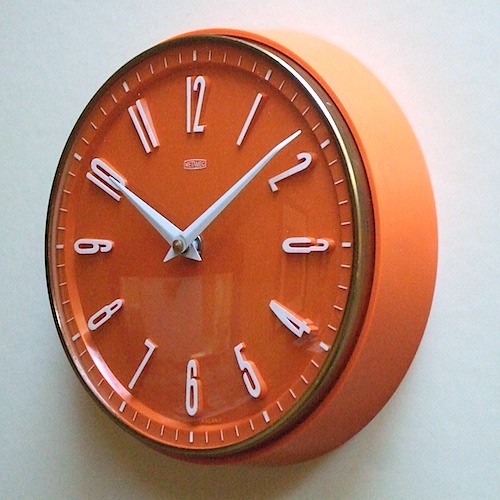On a light gray background, a strikingly unique clock is mounted on the wall. Dominating the scene, this large, thick, orange timepiece commands attention with its vibrant hue. The clock boasts a sophisticated gold rim encircling its face, adding a touch of elegance. The interior is a brilliant orange featuring precise, white minute markers and straight-lined, white numerals that are clear and easy to read. The long, pointed clock hands, also white, stand out against the bold background. Notably, the numeral three is distinct, resembling a zero more closely than a typical three, adding a quirky charm. At the top of the clock face, a small white square holds a word that is unreadable. This clock, with its blend of modern design and playful details, is both functional and visually appealing.